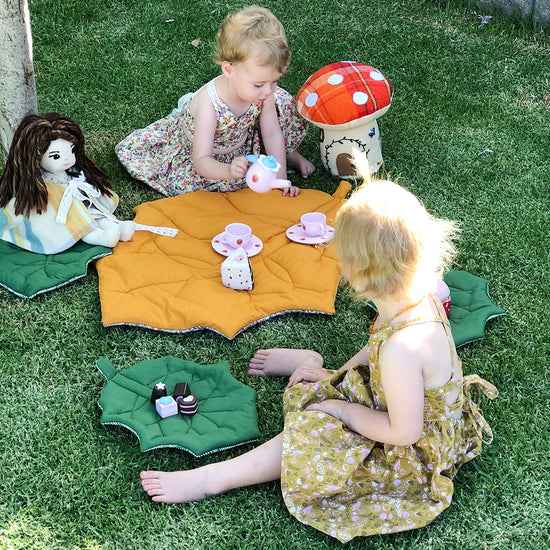In a sunny backyard, two blonde, Caucasian girls in floral sundresses are having a delightful tea party. They're seated barefoot on the lush, dark green grass, surrounded by an arrangement of fabric mats shaped like leaves. The largest mat, shaped like a gold leaf, acts as their table, adorned with two pink teacups and saucers, a pink teapot with a heart, and some pretend cakes and chocolates. Beside them, placed on smaller green leaf mats, are their dolls—one with long black hair and another brown-haired doll partially obscured behind one of the girls. A whimsical stuffed mushroom adds a touch of enchantment to their charming setup. The scene captures the joy and innocence of childhood, as the girls immerse themselves in the imaginative world of their tea party.